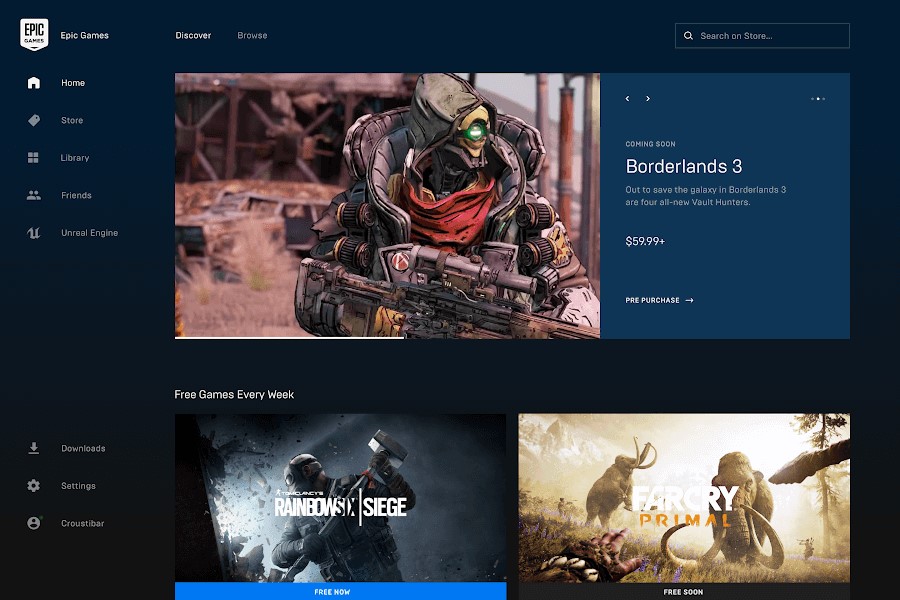Screenshot of Epic Games Store Interface:  
At the top, the prominent Epic Games logo is clearly visible. Below the logo are tabs labeled "Discover," "Browse," and "Search," with a magnifying glass icon representing the search function. The main navigation panel on the left side of the screen features options: "Home" (highlighted in white), "Store," "Library," "Friends," and "Unreal Engine". 

Central to the image is a highlighted promotional banner featuring the game "Borderlands 3" with an eye-catching graphic of a character in combat. The banner reads "Coming Soon: Borderlands 3" and includes the tagline "Set off to save the galaxy in Borderlands 3 with all-new Vault Hunters." The price is listed as $59.99, and arrow icons are provided for more information.

At the bottom of the screen, there are additional options for "Downloads" and "Settings." A profile icon, which appears to be linked to the user's account, is presented in what seems to be another language, resembling "crucifar."

Overall, the interface is sleek and well-organized, facilitating easy navigation and discovery of new games.